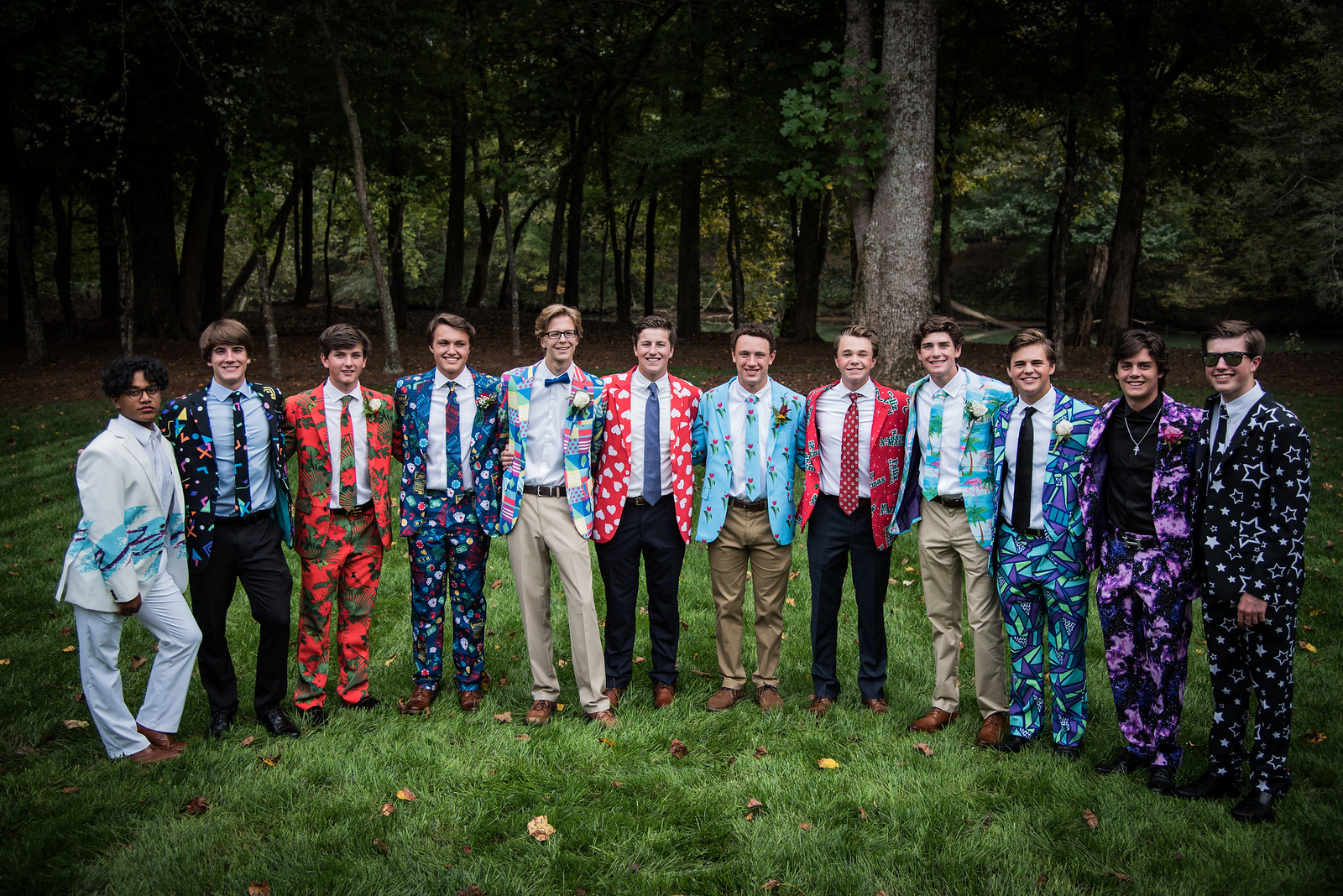In this vibrant and cheerful outdoor photograph taken on an overcast day, we see 12 young men aged approximately 15 to 21, standing in a slightly curved row on a lush, green grassy area, against a dense backdrop of tall, leafy trees. All the boys, who predominantly appear white with the exception of one boy on the far left who is of Hispanic or Mexican descent, are smiling warmly at the camera.

Each boy showcases a unique and brightly colored suit, suggesting a festive occasion, possibly prom. Starting from the left, the first boy, with brown skin, dark curly hair, and dark glasses, dons a striking white suit with blue and black zigzag patterns. Next to him, a taller boy with brown hair wears a vividly patterned jacket in reds, blues, and yellows, over a blue shirt and black trousers. The third boy, shorter with dark hair styled to the side, sports a red and green camouflage-style suit and a white shirt adorned with a carnation.

Moving along, there is a boy with brown hair, swept to the right, wearing a white shirt and a blue suit covered in bright circles of pink, turquoise, navy, and yellow. In the center, a tall man with glasses and a blue bowtie stands out in a jacket covered in various American state flags, paired with beige trousers. 

To his right stands a mid-height boy in a red jacket with white love hearts, a brown tie, black trousers, and brown shoes. Another young man, beaming broadly, is dressed in a turquoise jacket with roses, matching tie, beige trousers, and brown shoes. Continuing, we observe a boy with blonde hair, wearing a white shirt, red-spotted tie, and a red jacket, paired with black trousers and brown shoes.

Following him is a tall boy with dark hair, in a jacket featuring Hawaiian patterns, a white shirt, matching tie, beige trousers, and brown shoes. Next to him, a younger-looking boy with dirty blonde hair and a bright smile, wears a suit with purple, turquoise, and green stained-glass patterns, black shoes, and a black tie. 

On the far right, there is a boy with darker skin in a purple suit with smatters of pink and blue, wearing a black t-shirt and a necklace with a silver cross. Finally, the last boy, with dirty blonde hair and black sunglasses, stands out in a black suit covered in star designs over a pale blue shirt.

The overall scene is a captivating mix of colors and smiles set against the serenity of a forested background, capturing a moment of joyful camaraderie and style.